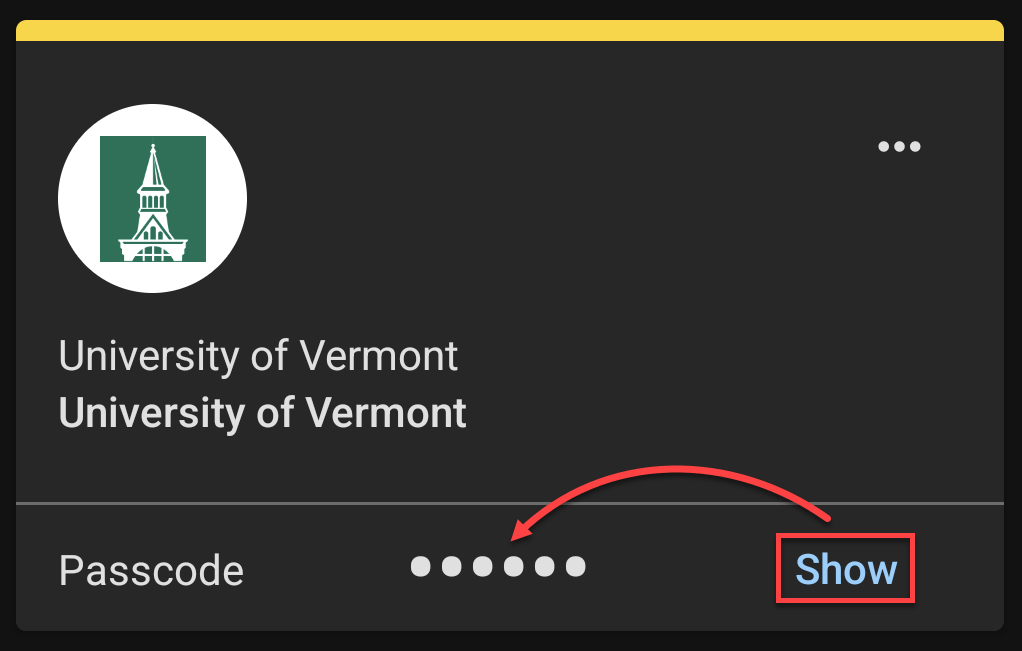This image depicts a zoomed-in section of a computer screen displaying a passcode entry field. At the top of the image, partially inset, is a yellow tab that is almost rectangular but features a curved top edge with a mustard-yellow color. Below this tab is the emblem of the University of Vermont, characterized by a circular seal. Within this circle, a green rectangle houses the distinctive, long, and skinny pointy roof of a campus building.

Directly underneath the emblem, the words "University of Vermont" are displayed twice; the second instance features a slightly thicker font. At the bottom of the image, "passcode" is written in white text. Below this, six dots represent the input for the passcode. To the right of this, the word "show" is enclosed in a red rectangle, indicating the option to display the passcode.